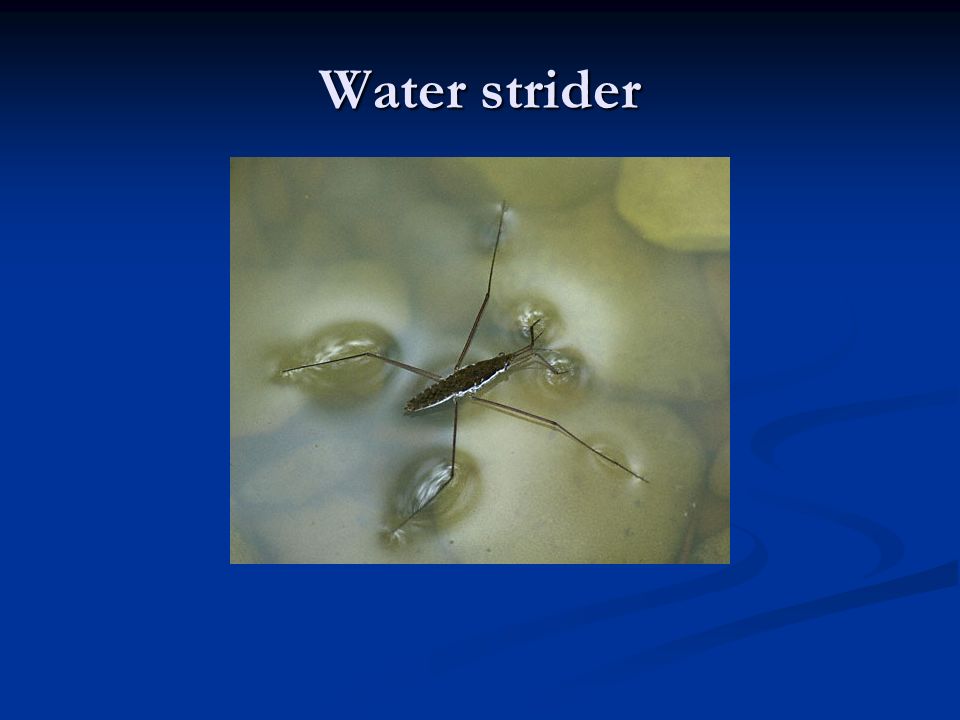The image is a detailed poster featuring a water strider, prominently displayed against a blue background. The background exhibits a dark cerulean blue color with additional wavy lines in a slightly darker shade decorating the bottom right corner. At the top, the blue deepens to a darker hue.

Centrally placed on this blue backdrop is a rectangular photograph of a water strider. The insect, characterized by its oval-shaped, brownish body with white trim, is shown resting on the surface of shallow, cloudy water. Its four long, thin legs and two antennae stretch out, causing noticeable surface tension where its legs meet the water, creating light reflections and curvatures around the displacement points. Despite the cloudiness, the water is shallow enough to reveal some round, gray stones lying at the bottom.

Above the insect within the framed photograph, the title "water strider" is written in white text, with the 'W' in uppercase and the rest of the letters in lowercase. The overall composition gives a detailed and scientifically intriguing depiction of the water strider on water, making it suitable for educational or presentation purposes.